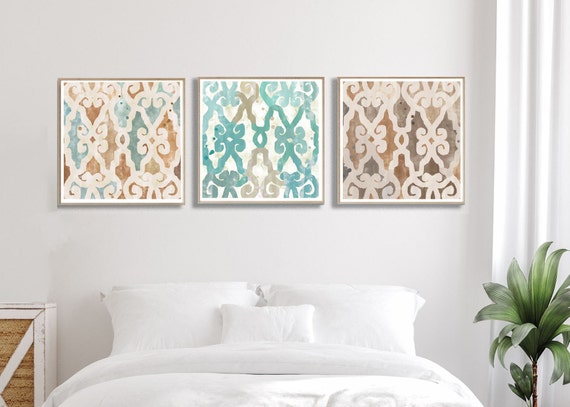The photo depicts a professionally styled bedroom, likely from a home decor magazine, filled with natural daylight. Central to the image is a well-made queen bed featuring a pristine white bedspread that is folded back near the headboard. Neatly arranged on the bed are two large pillows flanking a smaller throw pillow. The bed is set against a white wall, which has a vertical white panel extending from the top to the bottom, complemented by a soft lavender hue behind it.

Above the bed, three square paintings are evenly spaced, each showcasing unique designs but in cohesive colors. The left painting features light teal and brown hues, the center painting is more predominantly teal, and the right painting shifts towards brown with no teal.

To the right of the bed, a lush green plant with large leaves sits near a white drape, hinting at a window that streams daylight into the room, enhancing the tranquil ambiance. On the left side of the bed is a stylish nightstand with a white exterior and a brown wood interior, adding a touch of contrast to the room's airy and elegant aesthetic.